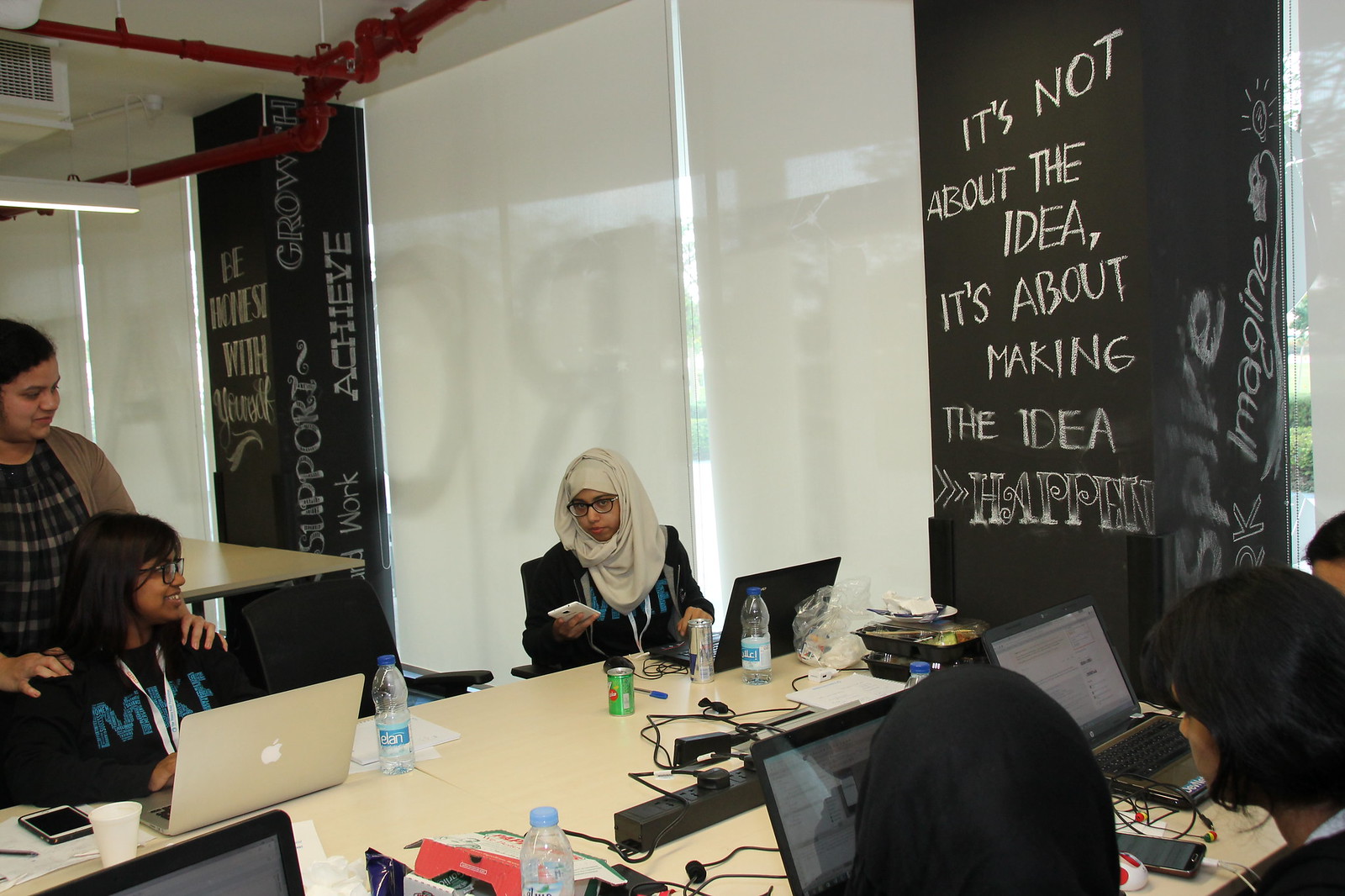In this vibrant and bustling study room, a diverse group of individuals, primarily of Asian descent, are seated around a large, light off-white grain table, engrossed in their work on various Apple laptops. The room is softly illuminated, with light filtering through white curtains that cover the windows. Dominating the right side of the room is a large black pillar adorned with motivational words written in chalk, prominently displaying the phrase, "It's not about the idea, it's about making the idea happen."

In the foreground, a Muslim woman with a round face and white hijab sits in front of her laptop, wearing glasses and engaged in conversation. Next to her, another woman is seated at an Apple laptop. She has dark brown hair, a black hoodie with a lanyard, and glasses with black frames. A clear plastic bag, a computer mouse, a white phone, a pen, a green can, a water bottle, and a Red Bull are strewn around her workspace. Standing behind her is yet another woman, with a brown open shirt layered over a plaid shirt. Her hands rest gently on the seated woman’s shoulders, adding a supportive touch.

The room has an inviting, collaborative atmosphere, enhanced by the presence of other individuals busily typing away on their laptops, with various beverages like water bottles and cans scattered across the table. It feels like a dedicated space for brainstorming and bringing ideas to life.